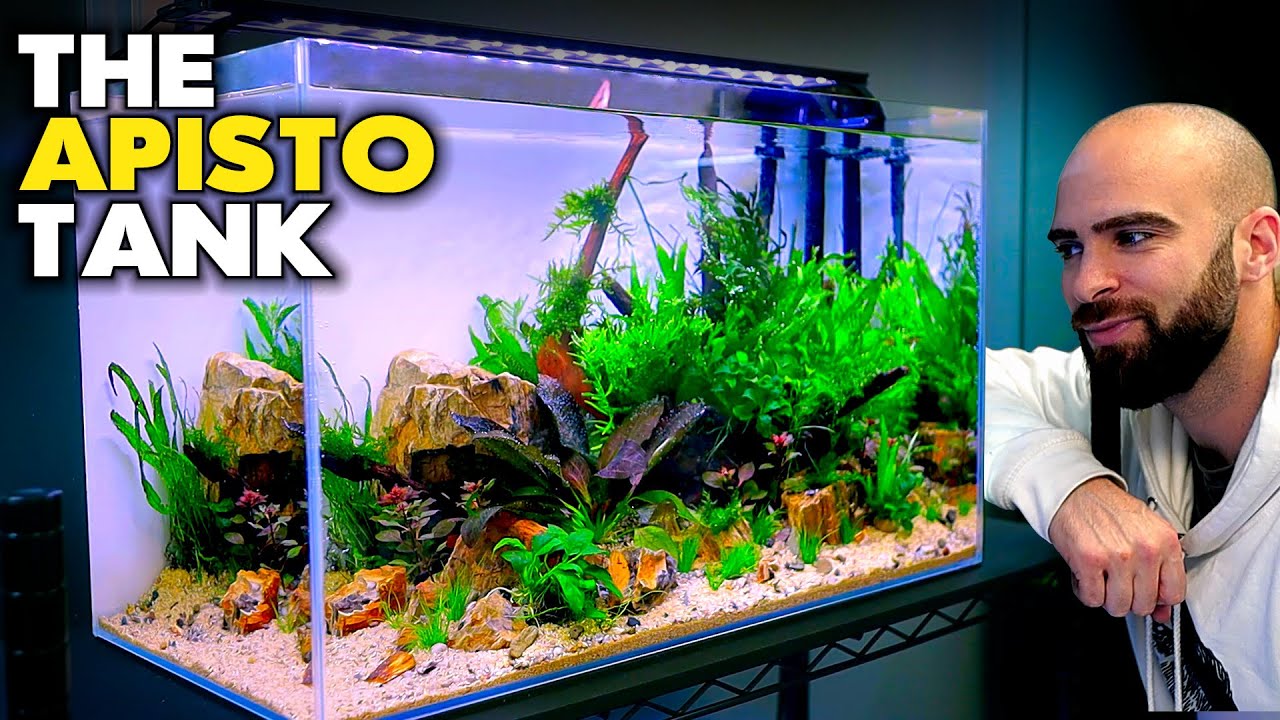In the image, a bald-headed man with a beard and mustache, wearing a white shirt or jacket, is intently observing a large, neatly arranged fish tank. The tank is housed in a dark cabinet, which might be black, and features metal accents. The background walls of the room are a greenish-blue hue. The fish tank itself is quite spacious, with a blue section at the top symbolizing the sky and clouds, and contains sand at the bottom along with a variety of plants and stones. The greenery includes both vibrant green water plants and darker, possibly purplish-colored leaves. There are several orange-hued stones and wooden elements, as well as a prominent large rock on the left side of the tank. At the top of the tank, text in white and yellow font reads "THE APISTO TANK". The man, appearing in his 30s or 40s, is leaning his arm on the cabinet and smiling, seemingly appreciating the setup of the aquarium.